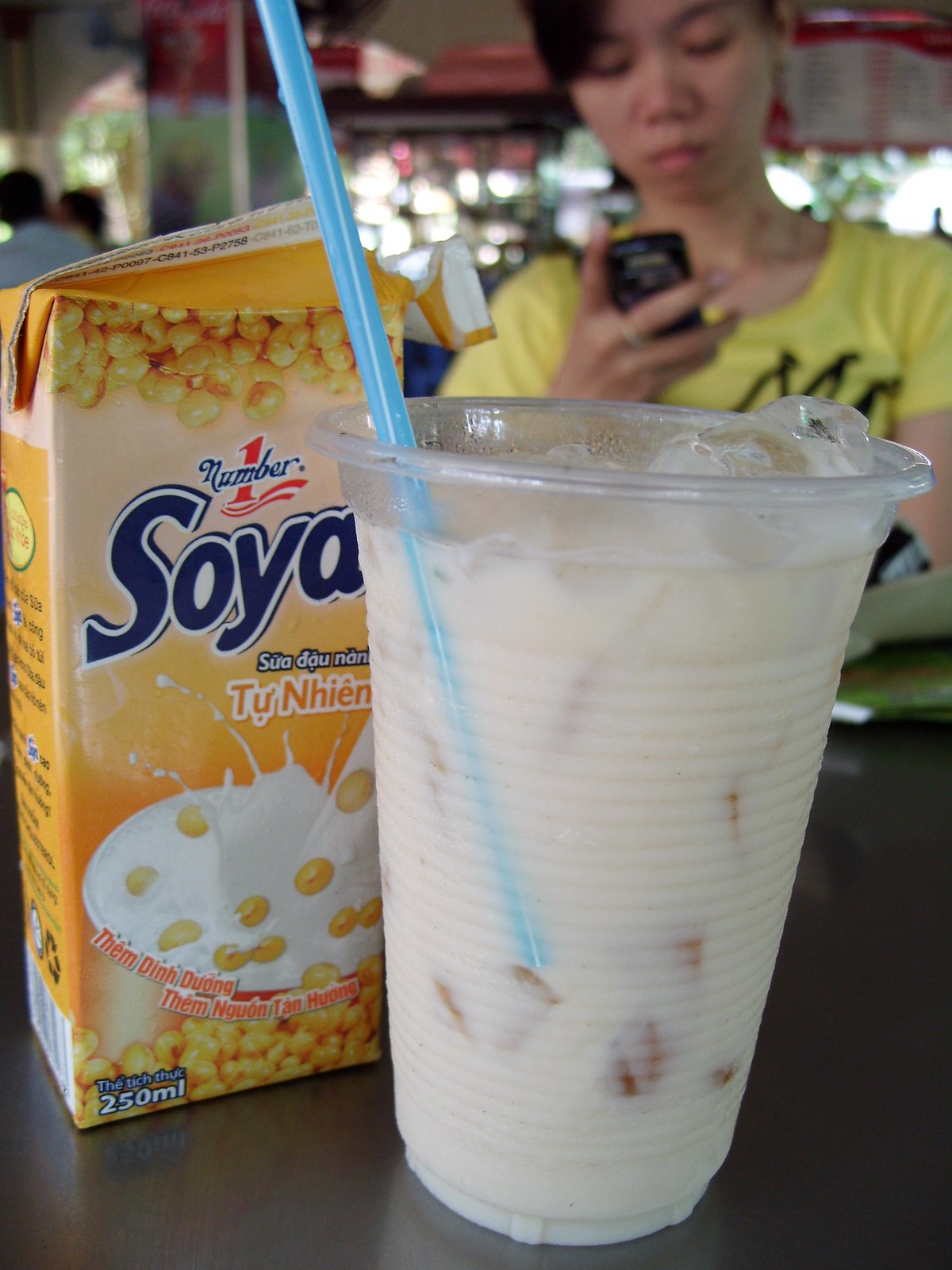This photograph captures an indoor scene, likely within a restaurant or café. Centrally placed in sharp focus on a table is a clear plastic cup containing a milky, iced beverage, presumably soy milk given the presence of a yellow carton labeled "soya" with both English and Asian writing, and depictions of soybeans. The beverage is chilled with clear ice cubes and features a sky blue plastic straw. Complementing the drink is a yellow cardboard box of soy milk that also includes soybeans in a bowl depicted on the packaging. In the background, slightly out of focus, is an Asian woman dressed in a yellow short-sleeved t-shirt with some black details, engrossed in her cellphone. The restaurant setting is softly lit, enhancing the ambient atmosphere, with additional patrons visible in the far background. The overall scene suggests a cozy moment capturing a popular Asian beverage.